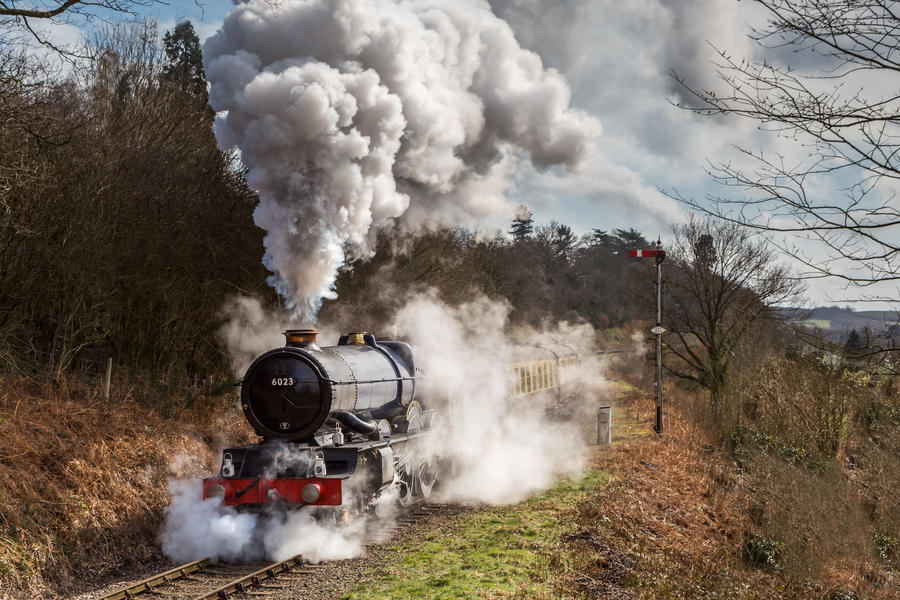The image portrays a steam engine train chugging forward amid a mountainous, barren landscape. The front of the train features a vivid red undercarriage, while the engine itself boasts a mix of black and silver. A voluminous plume of smoke billows from the top and sides of the engine, partially obscuring the train’s cars and the sky above, which is a faint blue scattered with clouds. The scene reveals a track cutting through a desolate countryside dotted with leafless trees, patches of dry grass, and dirt. A small, solitary pole stands to the right side of the track, hinting at an isolated rural setting.